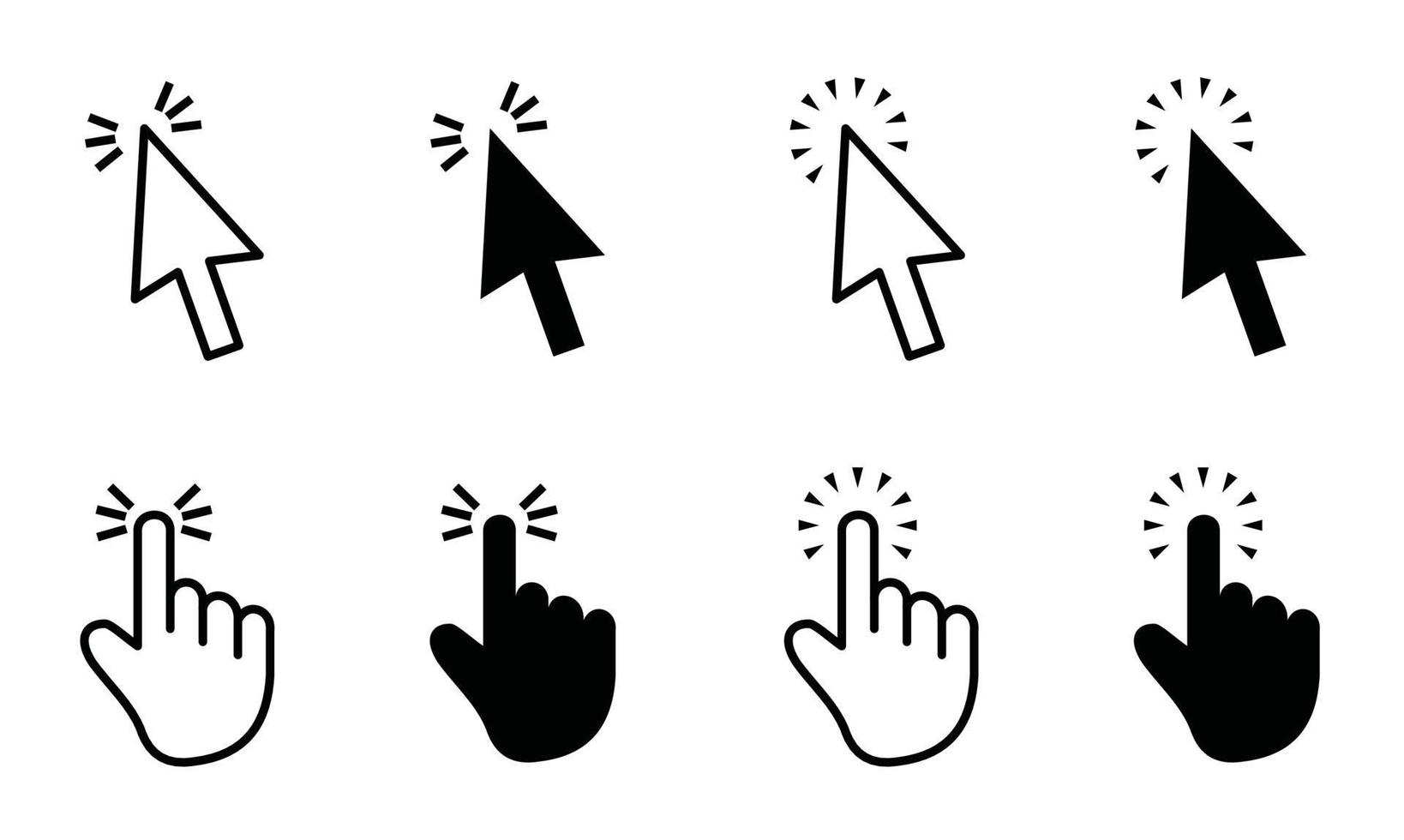This is a detailed black and white illustration of eight computer graphic icons representing various pointer emojis. The top row showcases four triangular arrow pointers, while the bottom row features four hand pointers with the index finger extended and thumb sticking out. Within each row, the pointers are displayed with alternating colors and effects. 

Starting from the left in the top row, the illustrations include:
1. A white arrow pointing up and to the left with small motion lines at the tip.
2. A black arrow in the same position with similar motion lines.
3. A white arrow pointing in the same direction, but with a pronounced halo effect around the tip.
4. A black arrow featuring the same halo effect.

In the bottom row, the hand pointers mirror the top row's sequence with corresponding colors and effects:
1. A white left hand with the index finger extended, showing small motion lines around the finger tip.
2. A black left hand in the same position with identical motion lines.
3. A white left hand, similarly positioned but with a halo effect around the finger.
4. A black left hand featuring the same halo effect.

The design alternates the color scheme both horizontally and vertically, providing a clear visual comparison between the different styles and effects of the pointers.